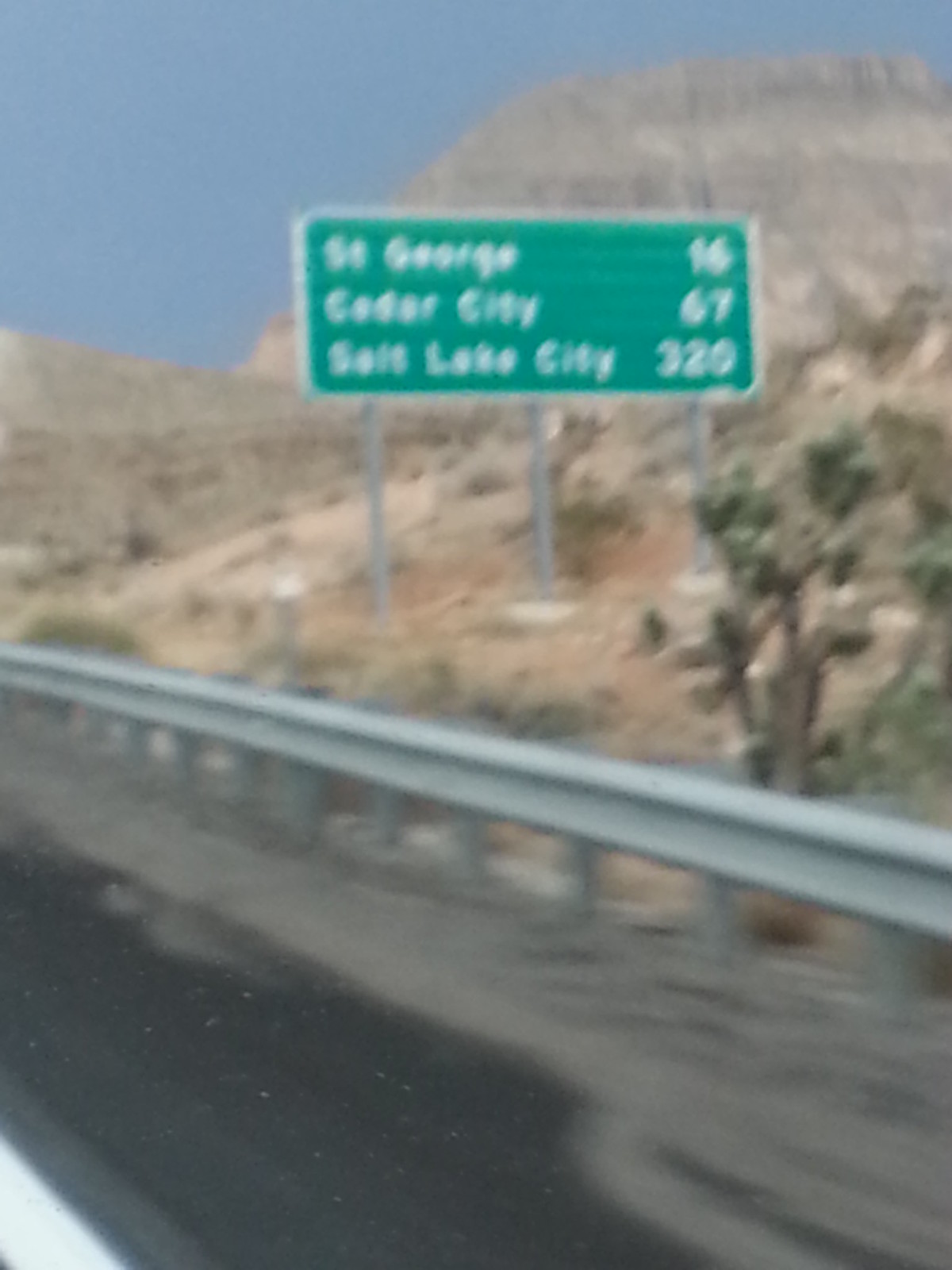This blurry, portrait-oriented image captures a highway scene dominated by a large green road sign centered in the upper portion of the frame. The rectangular, landscape-oriented sign is held up by three metal posts, and features white text and a white border. The sign provides mileages to various cities, reading "St. George 16," "Cedar City 67," and "Salt Lake City 320." The background behind the sign is a rugged, rocky landscape with sparse vegetation, characterized by a tan, sandy ground and a prominent rocky hill or mountain. The sky in the upper left corner is a clear medium blue with no clouds. In the right center of the image, there is a small, stubby tree with a brown trunk and green leaves, standing approximately four to five feet tall. Spanning across the middle of the image, a standard silver metal highway railing dips slightly as it extends from the middle left to the lower right. Below the railing is the gray shoulder of the highway, marked by a white line and partially obscured by a dark, almost black shadow suggestive of a passing vehicle. The overall setting is consistent with a desert-like environment, where the arid terrain and sparse greenery contrast with the structured elements of the highway infrastructure.